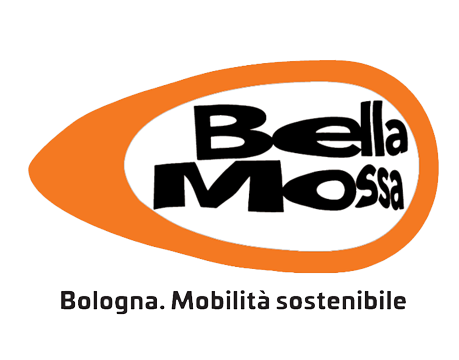The image depicts a minimalist logo set against a pristine white background. Central to the design is an orange, horizontally oriented oval or egg shape, with its narrower end pointing to the left and its broader section to the right. The orange shape frames an inner white section where the brand name "Bella Mossa" is prominently displayed in bold black text. Directly beneath this, in finer black print, are the words "Bologna Mobilita Sostenibili." The orange oval varies in thickness, approximately half an inch for most of its circumference and expanding to nearly an inch in one area, adding a dynamic flair to the otherwise straightforward design.